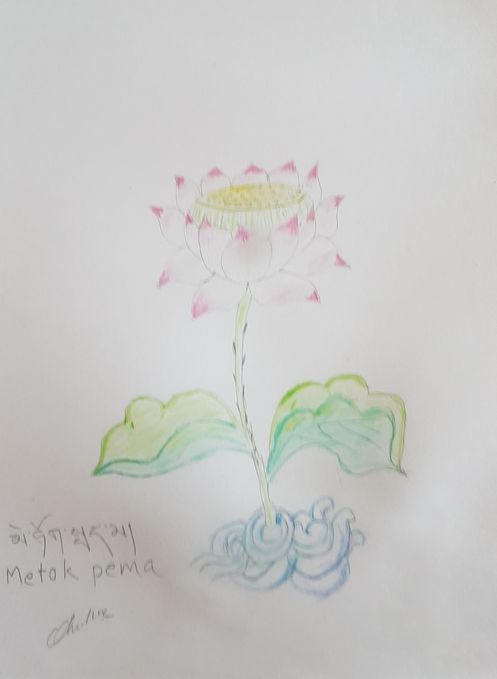This is a detailed colored pencil drawing of a vibrant flower, meticulously depicted with two distinct levels of petals. The inner layer of petals, closest to the center, stands upright while the outer layer gracefully curves downward. Each petal showcases a striking blend of pink tips and a harmonious gradient of pink and white hues. The flower’s center is adorned with a vivid yellow core, reminiscent of the dark center found in a sunflower.

Extending from the flower is a notably long stem that supports two intricately shaded leaves, displaying a captivating interplay of light and dark green tones at the base. Adding an intriguing element to the composition, the flower appears to be encircled by a chain at the bottom.

The artwork is centered on an 8 by 11 inch sheet of pristine white paper. In the bottom left corner, the artist, Mataka Purma, has signed her name in a unique fashion. The signature is rendered in three distinct styles: her native language script, English, and elegantly in cursive, adding a personalized and multicultural touch to the piece.